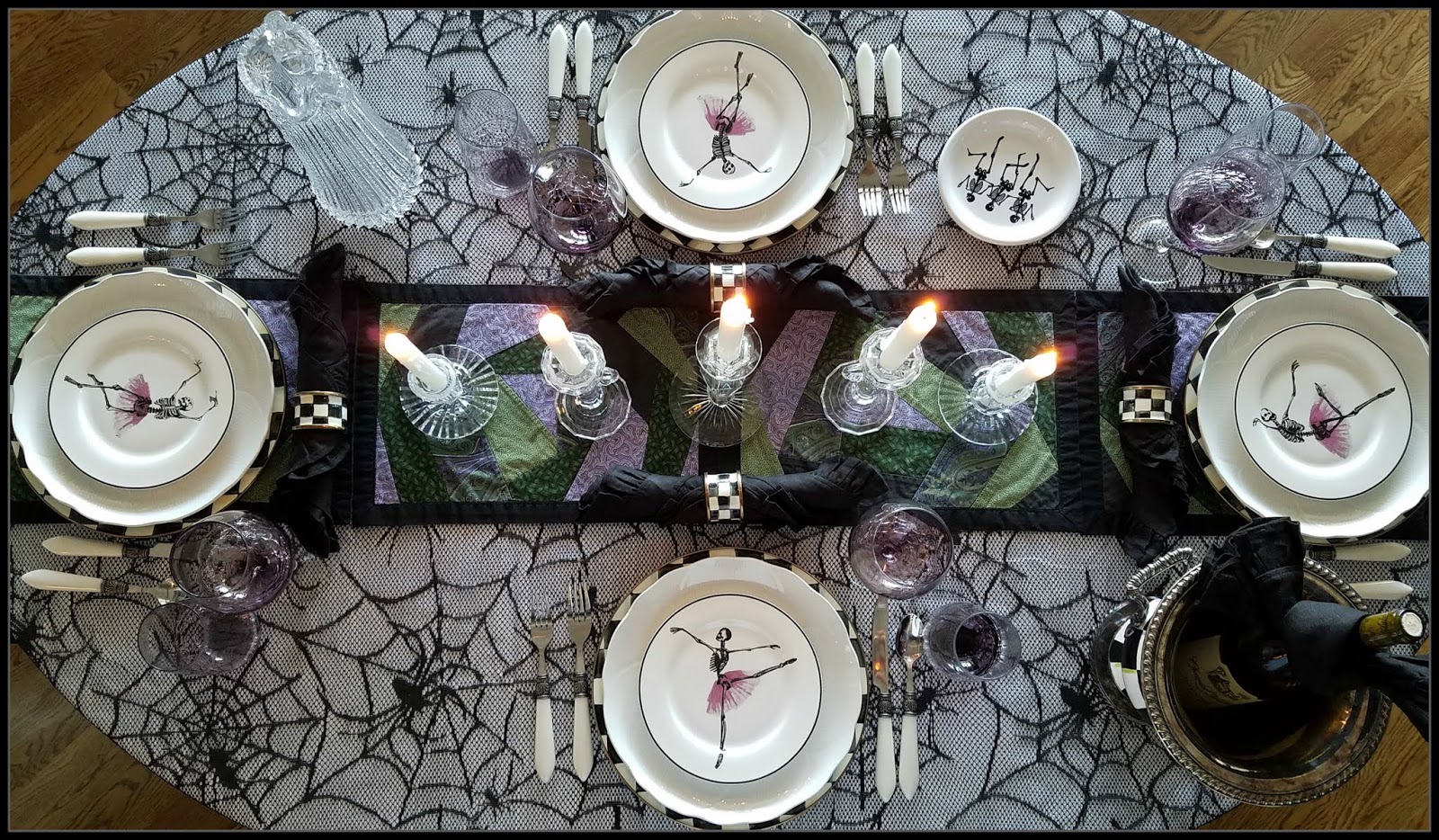This top-down photograph captures a gothic-themed Halloween table setting for four, with an intriguing blend of steampunk elements. The table features a large wooden surface covered with a light gray, oval-shaped tablecloth adorned with black spider webs and spiders. In the center, a vibrant table runner with geometric patterns in black, purple, blue, and green stretches beneath five lit white candles in glass holders.

Each place setting is meticulously arranged and unique, beginning with a black and white checkered bowl at the bottom, followed by a plain white bowl, and topped with a small plate depicting skeletal ballerinas in tutus. The cutlery is placed precisely with knives, spoons, and forks sporting silver and white, possibly porcelain, handles. Complementing the eerie aesthetic, each setting includes a purple glass, likely for wine, matching the gothic color scheme.

To complete the ensemble, there is a black and white checkered wine chiller, echoing the design of the bowls, housing a bottle of bubbly. Matching napkin rings also feature this checkered pattern. Additionally, the table includes a water jug, much needed amidst the hauntingly beautiful decor.